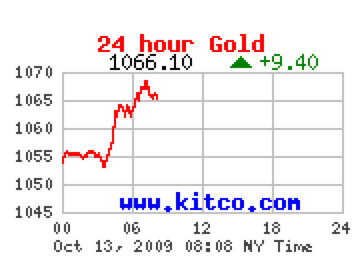The image depicts a detailed line graph illustrating the movement of gold prices over the last 24 hours. At the top of the graph, in red font, it reads "24-hour Gold." Directly beneath this, in black text, it displays the current price of gold as $1,066.10, accompanied by a green upward arrow indicating a rise of $9.40. The vertical axis on the left side of the chart represents the price range of gold, marked from $1,045 to $1,070 in increments of 5. The horizontal axis at the bottom is labeled with time intervals, starting from 00 and increasing in increments of 6 up to 24, showcasing a full day's movement. The chart prominently uses a color scheme of white, black, red, green, and blue against a black background. A red line traces the gold’s upward trend across the graph. The web address www.kitco.com is noted in blue text, indicating the source is a financial services website that focuses on commodities. Additional details at the bottom note the graph's timestamp as October 13, 2009, at 8:08 AM, New York Time.